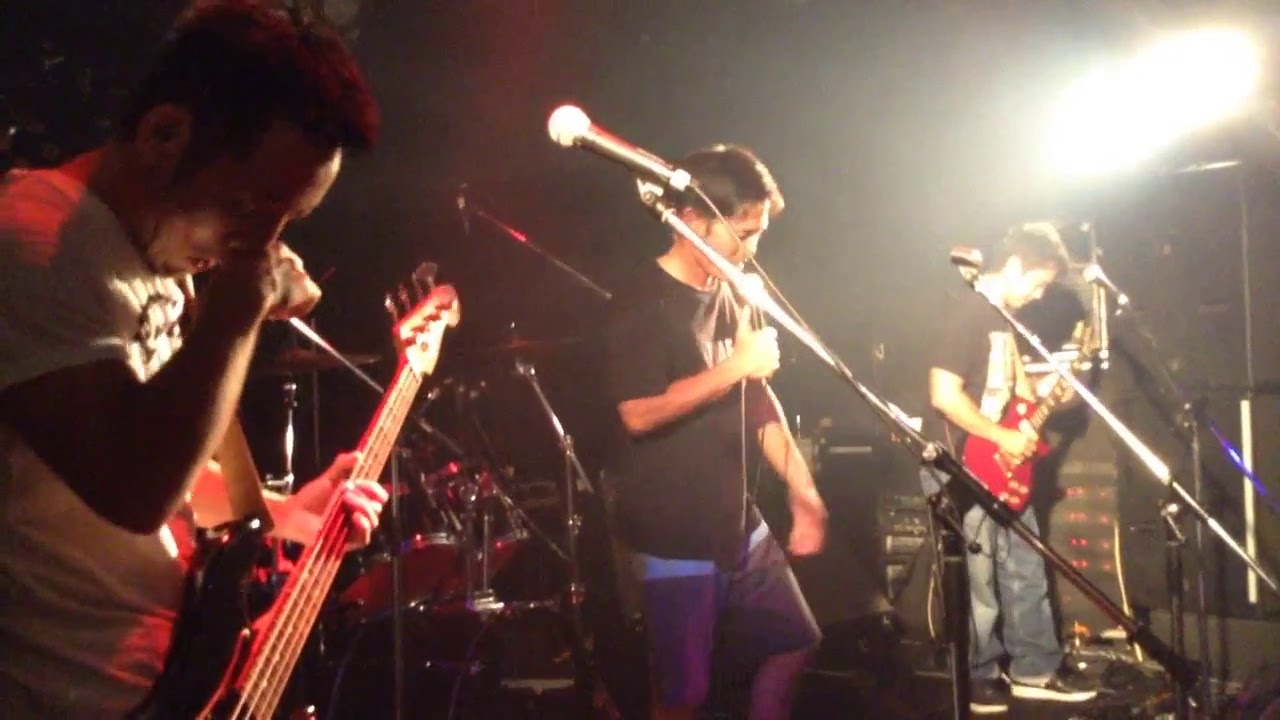The image features an indoor stage setting where a rock band is performing, illuminated by a single, intense light source from the upper right corner. This bright light casts stark shadows, highlighting the band members' faces and creating a dramatic ambiance against the otherwise dark and somewhat foggy background.

In the foreground, three male band members with short dark hair are lined up in a row, heads bent down and intensely focused on their instruments and performance. On the left, the guitarist with brown skin, wearing a short-sleeved white t-shirt and jeans, is holding his instrument with one hand while the other appears to be near his face. The lead singer, positioned in the middle, has short dark hair, brown skin, and is dressed in a black short-sleeved t-shirt and blue shorts. He is gripping the microphone stand and singing passionately into it. To his right, another guitarist, dressed in a black t-shirt with white print and blue jeans, holds a red guitar and is also looking downward.

Behind these three, partially visible in the darkened background, is a red drum set, though the drummer himself remains out of sight. In addition to the lead singer’s microphone, several other microphones on stands are visible around the band to capture their performance. The overall scene evokes a moody and engaging atmosphere typical of an indoor rock concert.